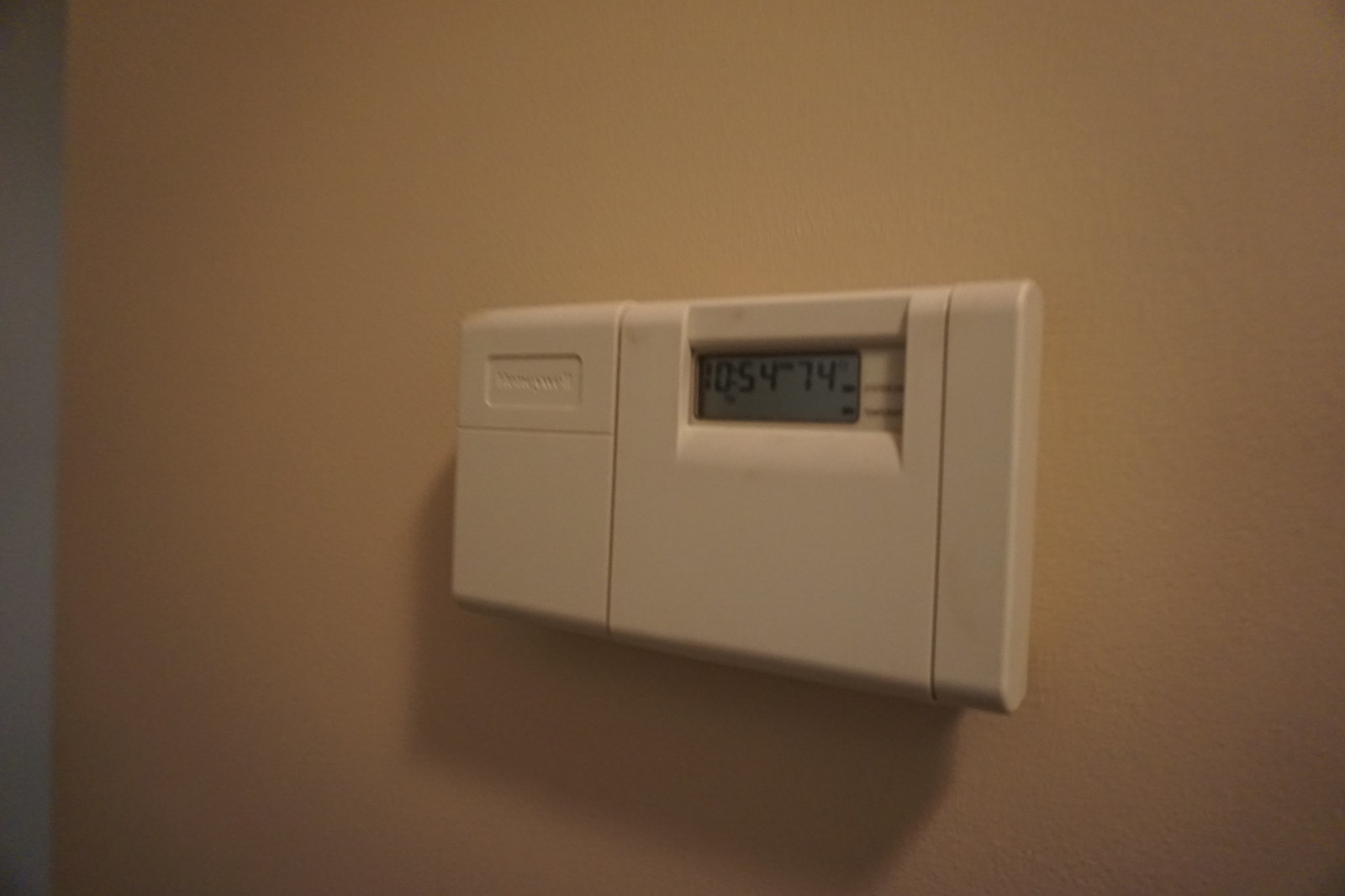This photograph captures a thermostat panel affixed to a light beige or pale brown wall. The wall corner is visible on the left side, creating an angled view of the panel that makes the left side appear slightly smaller than the right. The panel is a light, creamy beige color and features detachable components on the left side, likely for battery access. The upper right section of the panel houses a small digital display with a faint blue-gray background, displaying black text that reads "10:54 AM" and "74°F," indicating it functions as a thermostat.